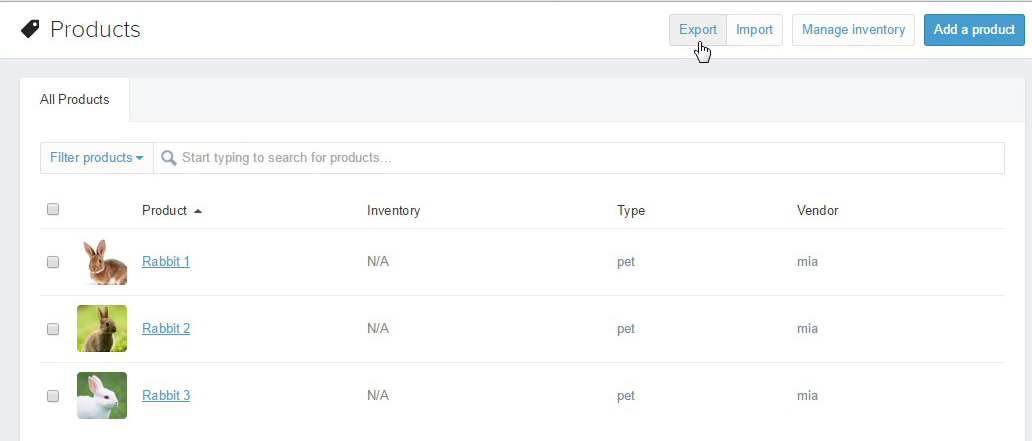In the upper left corner of the image, the word "Product" is written in black text on a black tag. The top right section features four tabs labeled "Export," "Import," "Manage Inventory," and "Add a Product." The "Add a Product" tab is displayed in white text on a blue background, while the other three tabs are written in blue. A white hand-shaped cursor hovers over the "Export" tab.

On the left side, a header reads "All Product." Below this, blue text says "Filter Product," and adjacent to it on the right is a search bar with the placeholder text, "Start typing to search for product." Beneath this section is a table with four columns: the first column is "Product," the second is "Inventory," the third is "Type," and the fourth is "Vendor." Each product listed is of the type "Pet," and the vendor for all is "MIA (M-I-A)." The inventory count for all products is not available. 

The products listed in the table have their names written in blue. The first product, "Rabbit 1," has an accompanying image of a brown rabbit with some white fur. The second product, "Rabbit 2," shows a completely brown rabbit against a green background. The third product, "Rabbit 3," features a white rabbit also set against a green background.